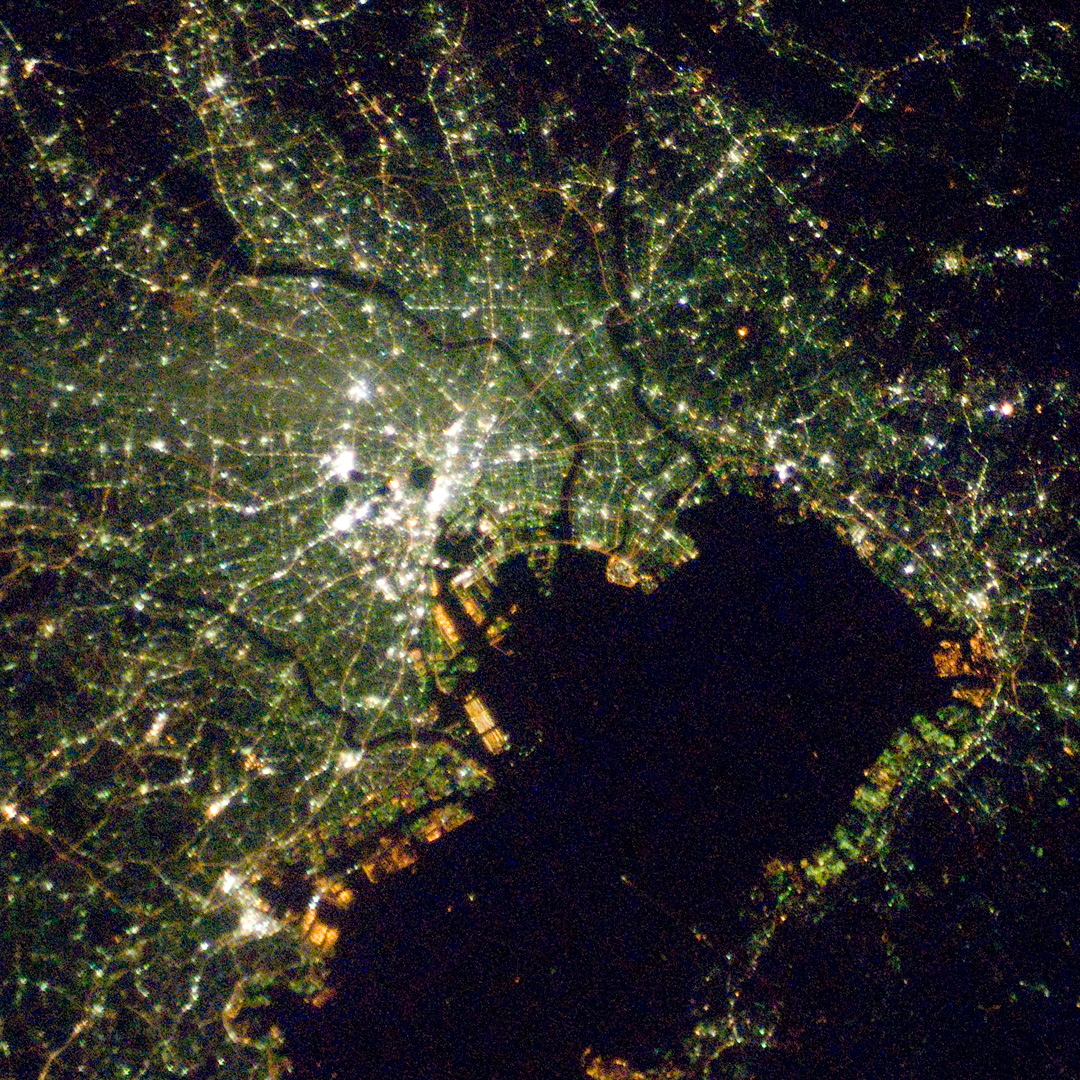This image is a highly detailed, aerial nighttime view of a large body of water bordered by land, resembling a strikingly complex circuit board. The perspective is from thousands of feet above, offering a broad overview. The scene is illuminated by a multitude of lights outlining the urban areas, roads, and state borders. There's a significant black area representing a body of water, possibly crossed by platforms. On the left side and the top, you can see distinct rivers adding to the city's layout. Scattered patches of green grassland are visible despite the overwhelming presence of artificial illumination, capturing the mixed landscape of nature and human development.